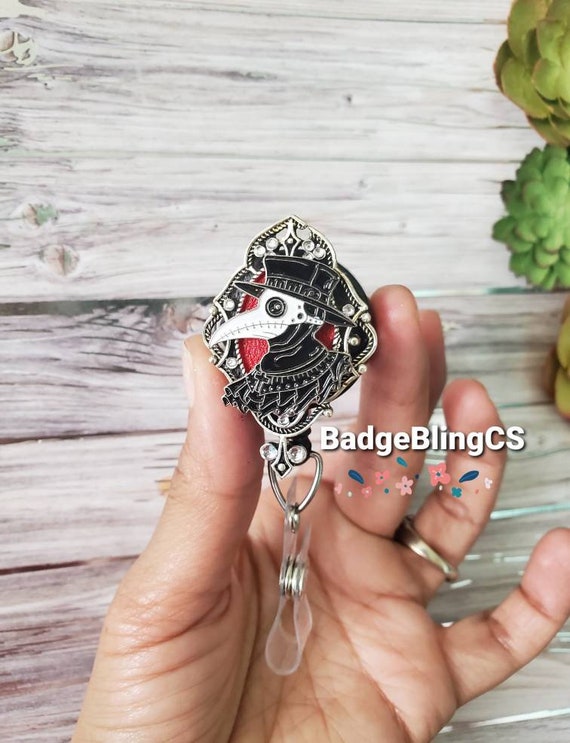The image depicts a hand holding a detailed and ornate keychain badge from a company called Badge Bling CS. The centerpiece of the keychain is an intricate design of a plague doctor mask, characterized by its bird-like beak, black hat, and stark white mask featuring a black, round eye. The badge is surrounded by fake diamonds, giving it a "blinged out" appearance. It features a ring at the bottom connected to a snappable lanyard for convenience. The badge also shows a portion of the figure's black, garnet-like attire, capturing the bust of the bird-like, skeleton-themed character. The background consists of a wooden fence with some succulents to the right-hand side, and beneath the product name "Badge Bling CS," there is a small spray of drawn flowers, likely part of the company's logo.